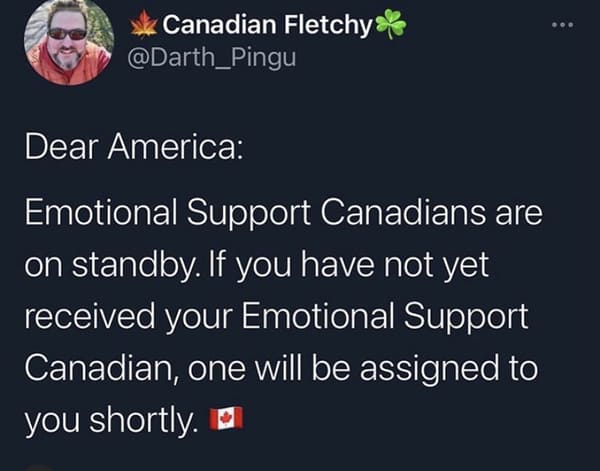The image is a screenshot of a social media post. At the center of the post, there is a circular avatar image depicting a selfie of the account owner. The individual appears to be a white male with short hair and a scraggly beard. He wears sunglasses and a heavy jacket, suggesting he is seated outdoors. His social media handle is "Canadian Fletchy," accompanied by a maple leaf and a three-leaf clover, which may represent a shamrock. Additionally, his username is displayed as @Darth_Pingu. The post has a black background with white text that reads, "Dear America, emotional support Canadians are on standby. If you have not yet received your emotional support Canadian, one will be assigned to you shortly." This message is followed by a Canadian flag emoji.